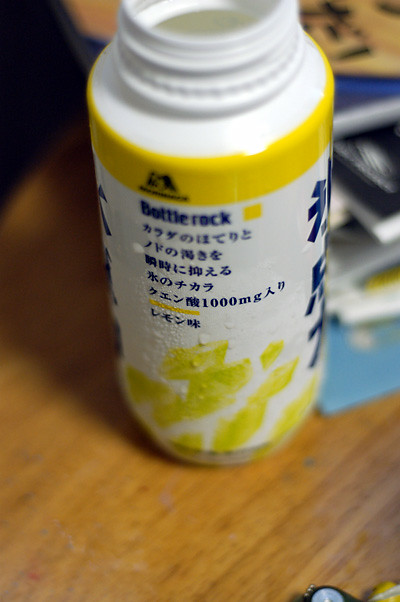An out-of-focus photograph depicts an empty white plastic bottle without its cap, resting on a wooden grain table. The top of the bottle is visible, showing a shiny white and yellow label slightly moist from condensation. The label features the text "Bottle Rock" alongside several rows of somewhat blurry Asian characters, with one row appearing sharper. Below this, it indicates a dosage of "1000 MG" amidst a pattern of yellow splotches. A yellow ring encircles the neck of the bottle. In the background, the table is cluttered with indistinct papers and books, adding context to the scene's setting.